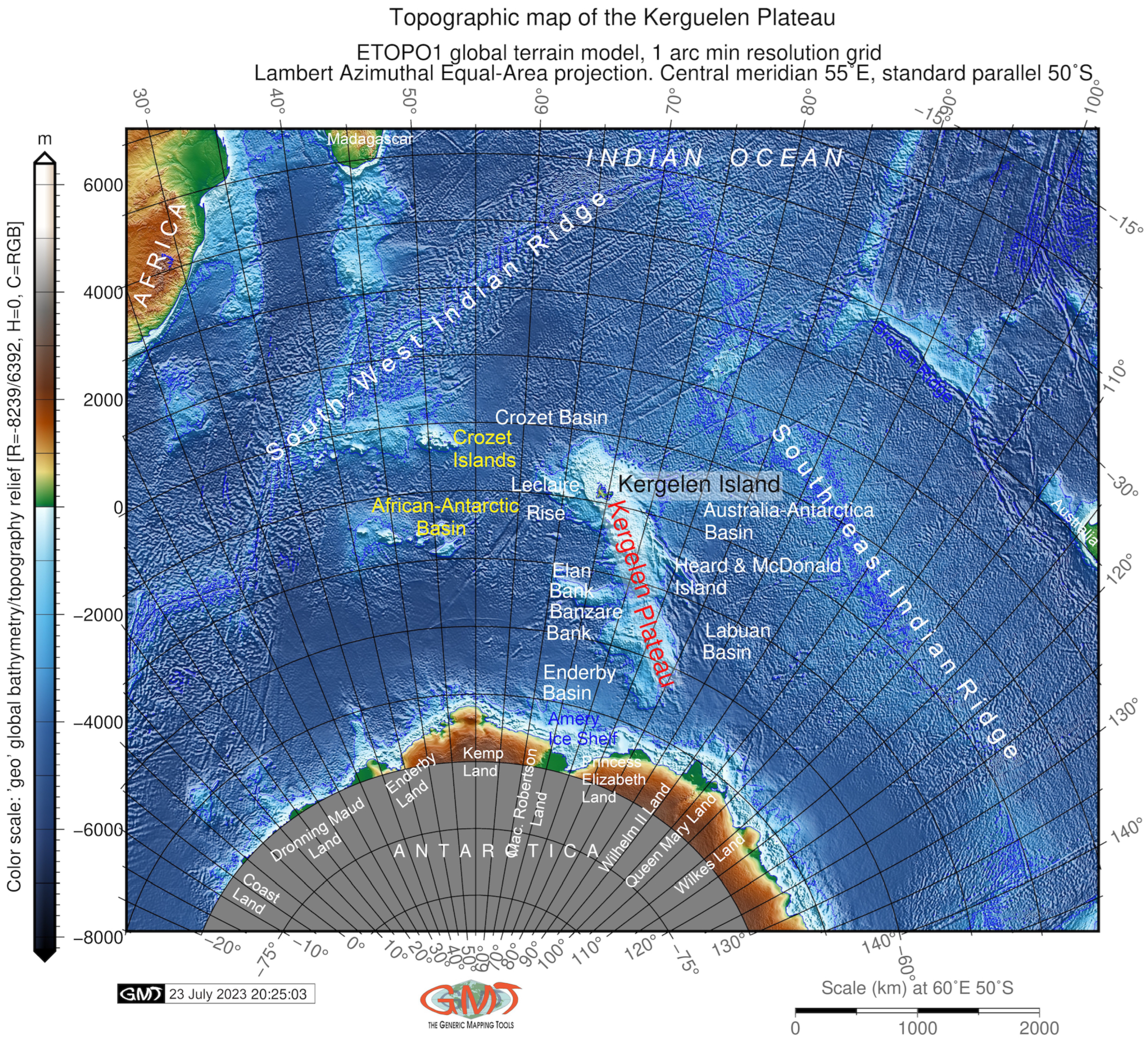The image is a highly detailed, square-format, computer-generated topographic map in color, depicting the Kerguelen Plateau and surrounding regions. Marked at the bottom with the timestamp "GMT, 23 July 2023, 20-25-03," it uses a Lambert Azimuthal Equal Area Projection with a central meridian at 55 degrees east and a standard parallel at 50 degrees south. 

The map is bordered at the top by a legend that reads "Topographic Map of the Kerguelen Plateau, ETOPO1 Global Terrain Model, 1-Arc Min Resolution Grid." The visual display emphasizes variations in elevation under the sea, showing valleys, peaks, and troughs with a color gradient: the ocean is primarily blue, darkening to deep blue along sub-ocean ridges like the South Indian Ridge and Southwest Indian Ridge, and lightening to white on the slopes. The landmasses are depicted in green and brown.

Antarctica is visible at the map's bottom, while the Indian Ocean is labeled at the top. Included are small sections of the eastern coast of Africa, Madagascar, and various islands such as Kerguelen Island, Heard, and McDonald Island. The Kerguelen Plateau itself is prominently labeled in red. The map is enriched with a color and numerical scale denoting bathymetry and topographic relief, offering a comprehensive view of submarine and terrestrial landscapes.